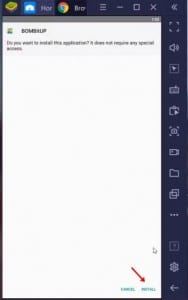The image quality is extremely poor, making it difficult to discern details clearly. In the upper left corner, there appears to be a green rectangular or square icon on top of a yellow one. To its right is a blue icon featuring what seems to be a white "home" button. Next to these is the recognizable Google icon, a circle segmented with red, yellow, and green, and a blue center.

This row of icons is set against a black strip running across the top of the image. There is an additional black strip on the right-hand side containing more icons: a sound icon, a square with an indeterminate symbol inside, a clipboard-like icon, a file icon, an icon of one square on top of another square, three vertically aligned dots, a settings gear icon, and a backward-pointing arrow.

At the very bottom of the image, two words are written in green, accompanied by an arrow pointing towards the word closest to the bottom right corner, though the text is indiscernible due to the poor resolution.